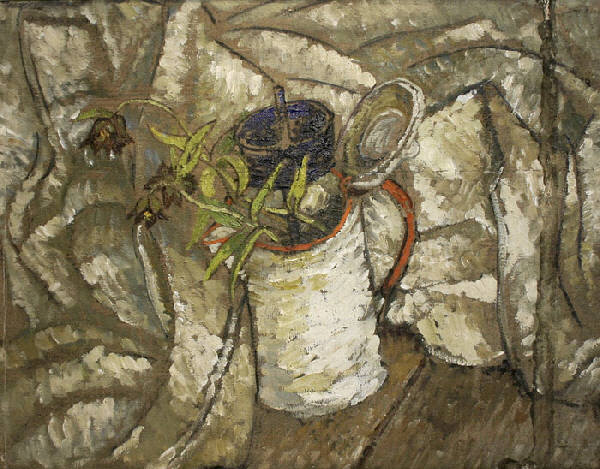This horizontal rectangular painting, predominantly rendered in shades of brown, beige, tan, and taupe, depicts a rustic scene set against a backdrop of wooden floor planks. Central to the composition is an intriguing canister, resembling a beer stein or coffee mug, which is cylindrical and primarily white with a defining dark brown handle. The lid of the canister is open, revealing a vibrant green plant emerging from within. Despite the plant's overall liveliness, some flowers droop with a brown hue, suggesting they are wilting. Surrounding the canister are several canvas bags or sacks, haphazardly piled in one corner, adding to the image's rustic charm. A wooden pole on the right side seems to support a possible shelf, contributing to the room's structure. Additionally, a subtle light source, possibly sunlight, illuminates the scene, hinting at natural light entering the space.